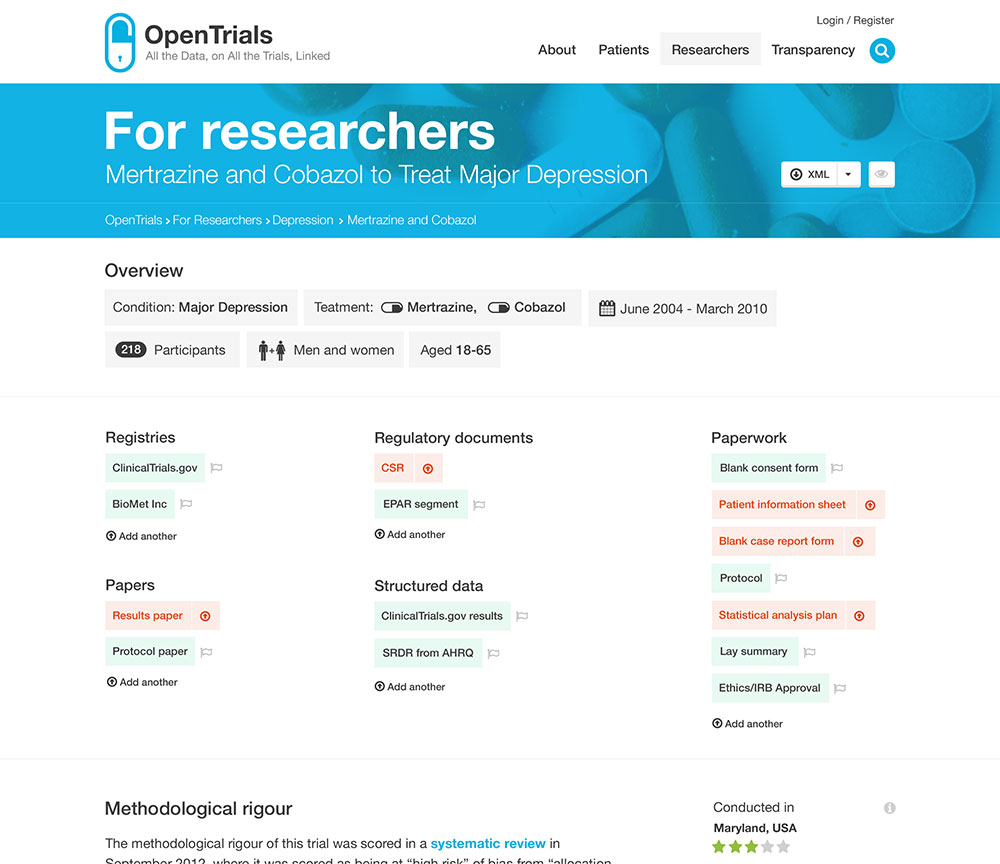The image displayed is a detailed view of a medical research website interface. At the top left corner of the interface, the website logo reads "Open Trials" in black text. Directly beneath it, there is a tagline stating "All the data on all the trials linked." Adjacent to this logo on the left side is a pill-shaped lock icon.

On the top right corner of the interface, there are options for user account actions, including "Login" and "Register." Just below this section, the website offers four navigation choices: from left to right, they are "About," "Patients," "Researchers" (which is currently selected), and "Transparency."

Dominating the middle portion of the interface is a large, blue rectangular box designed for researchers. The left side of this box prominently displays the title "For Researchers." Below this title, specific details about a study are noted, highlighting "Metronized and Cobasal to treat major depression." On the far right of this rectangle is a small label reading "XML."

In the central portion of the image, towards the top left, there is a heading that says "Overview," followed by a list of categories under it, including "Condition," "Treatment," "Participants," "Men and Women," and "Aged." At the bottom of the interface, there are additional categories such as "Registries," "Regulatory Documents," "Paperwork," "Papers," and "Structured Data."